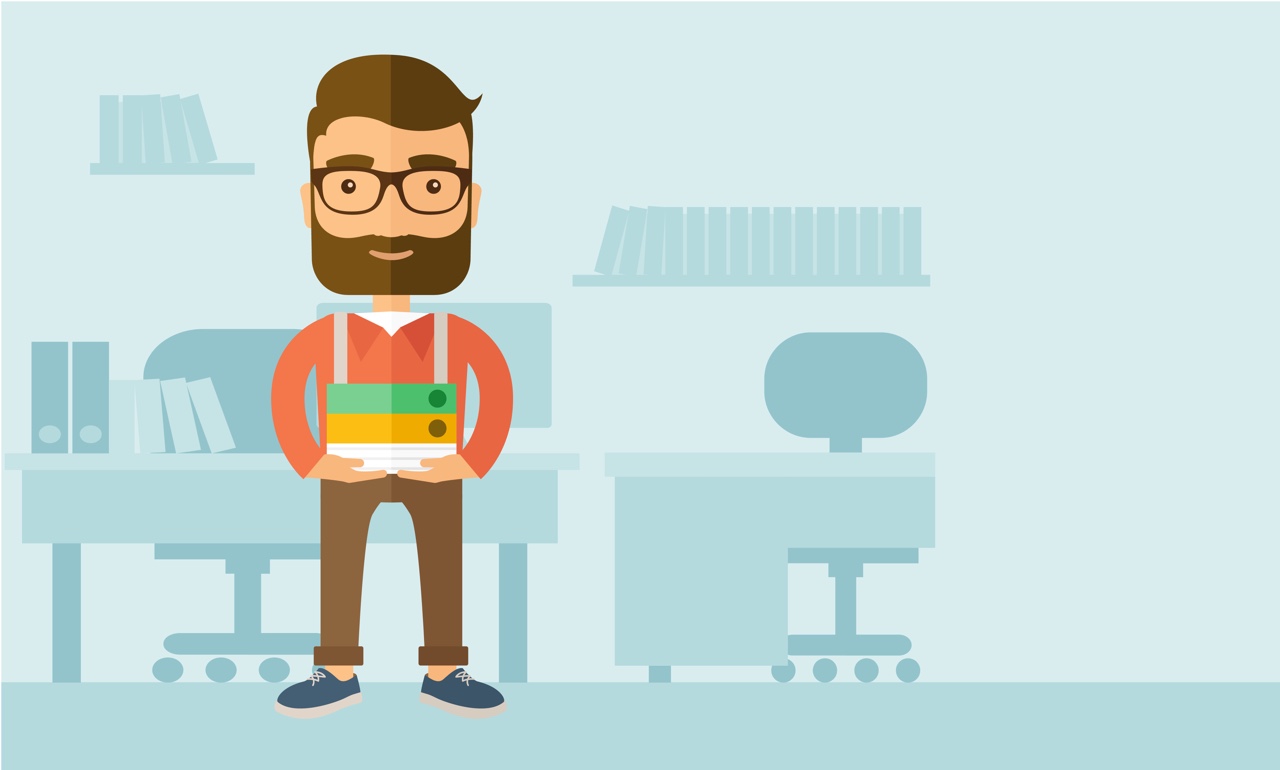This computer-generated, horizontally rectangular image features a stylized, cartoon-like man standing slightly left of center, in front of a lightly colored blue background. The background scene, illustrated in various shades of light blue, depicts an office or library setting with two small desks, chairs with wheels, and book-filled shelves. Everything in the background blends seamlessly together due to the uniform light blue coloration.

The man, prominently placed in the foreground, has short, wavy brown hair, thick brown eyebrows, and a full brown beard and mustache. He is wearing black-rimmed glasses that frame his black eyes. His attire includes a long-sleeved orange shirt with a collar, layered over a white t-shirt, brown pants, and blue tennis shoes with white laces and soles.

Held in front of him with both hands is a stack of three books. The top book is green, followed by a gold one, and the bottom book is white, each featuring holes on the right side. Unlike the monochromatic background, the man and the books he carries stand out with vivid detail and colors, drawing the viewer's attention to the central figure amidst the abstract office setting.